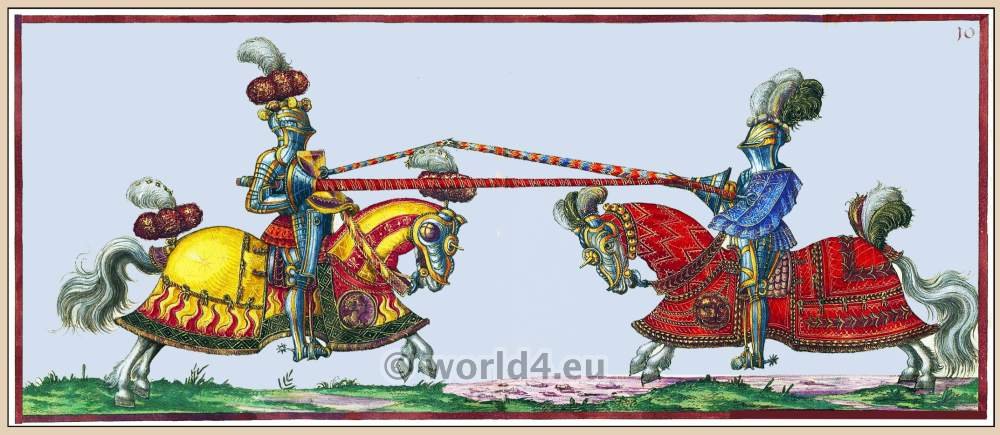This vintage image, marked with a "world4.eu" watermark in the lower fifth and numbered "10" in the upper right corner, depicts a detailed drawing of two knights engaged in a joust. The rectangular, horizontally oriented image showcases the knight on the right riding a gray horse draped in an ornate red cloak, complete with armor on its head. This knight wears a blue tunic over chainmail and a helmet adorned with feathers. His lance features red and blue stripes. Facing him on the left is another knight on a horse draped in a yellow and red ornate cloak. This horse also has armored headgear. The knight on the left dons a full metal suit with chainmail, a helmet with feathers and fur, and his red lance pointed towards his opponent. Both knights and horses feature intricate details, embodying the grandeur of medieval jousting tradition. Additionally, there are two insignias present in the image, one on each side, each displaying the face of a ruler, resembling coins.